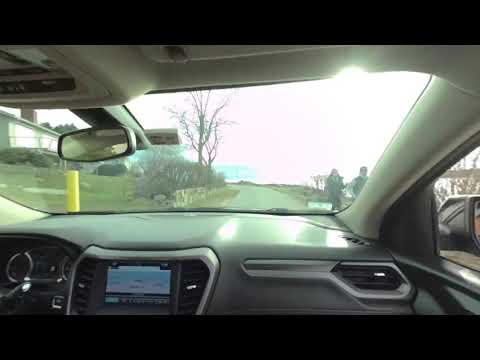The photograph is taken from the passenger seat of a modern car with the steering wheel on the left, providing a view through the windshield and part of the passenger window. The interior features a gray and light silver dashboard, with a central heads-up LCD display and a rearview mirror visible. The A-pillars are white, and the roof is light gray. Outside, a bright, sunny day illuminates the scene, with the sun shining through the top right corner of the windshield. The road ahead splits green grassy areas to the sides, with some trees and bushes, barren of leaves, on the left. There's a house visible on the far left beyond the lawn and buildings. On the right side of the road, two pedestrians are walking near what appears to be a potential cliffside. A yellow pylon, a stone-like wall, and additional structures are discernible in the surroundings.